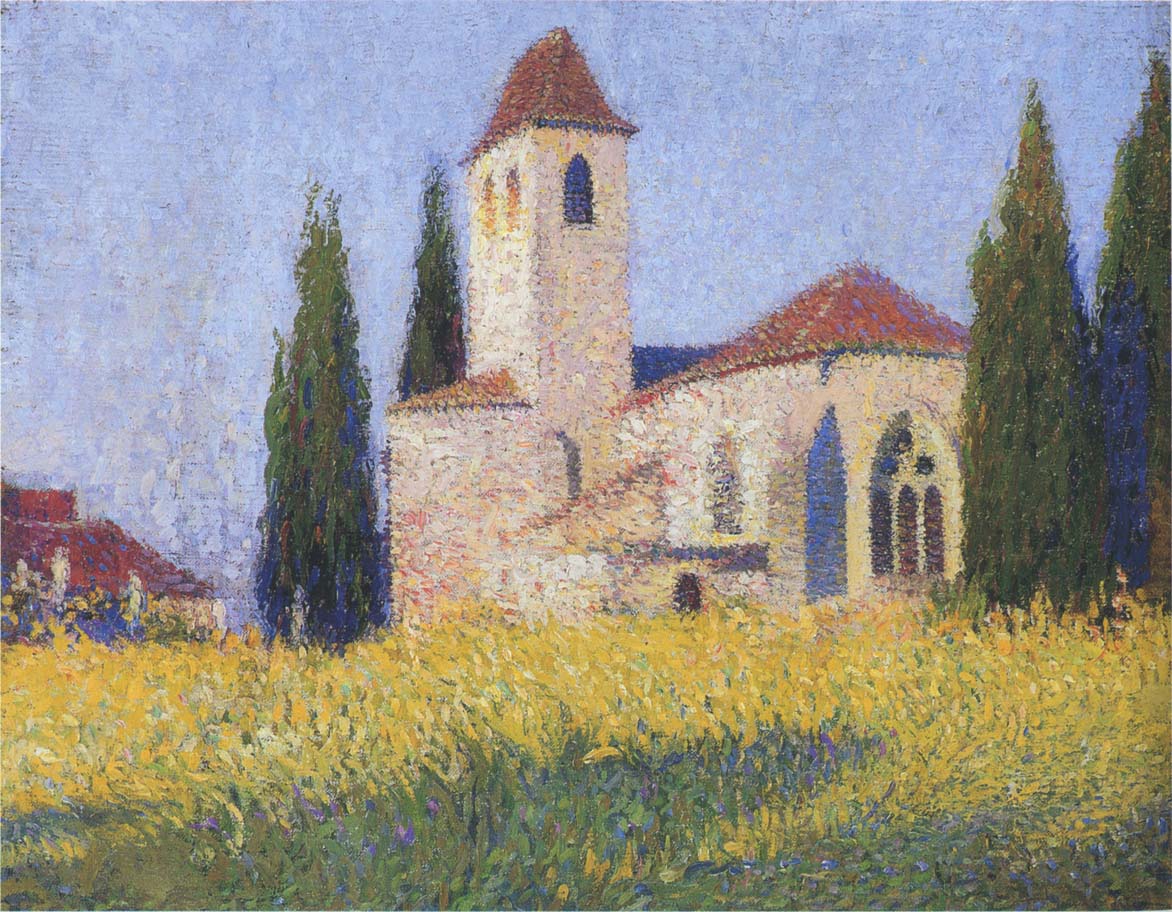This painting, possibly reminiscent of Van Gogh's style, depicts a historic church set slightly off-center to the right against a light blue sky. The church features a striking white facade complemented by a darker reddish-brown tiled roof. A prominent tower, akin to a steeple, is visible on the left side and shares the same red roof. The church's many arched windows and doors add to its traditional aesthetic. Tall, slender evergreen trees flank both sides of the church, enhancing the serene atmosphere. In the foreground, a lush field of long, flowery grass stretches out, adorned with yellow flowers and occasional hints of purple blossoms. On the left-hand side, partially obscured, lies another building with a similar red roof, suggesting an old-fashioned architectural style continues throughout the scene.